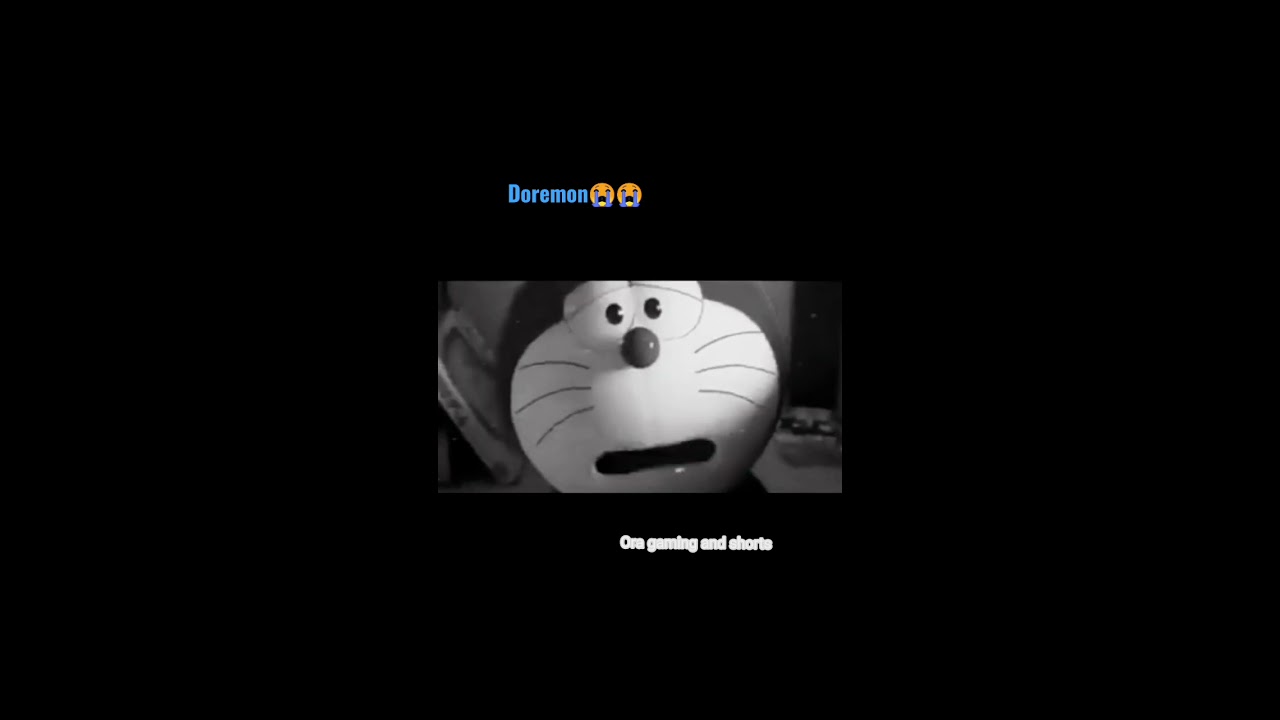The image is a wide rectangular digital artwork with a predominantly black background. Centrally positioned is a small, wide rectangular depiction of a cartoon animal, which appears to be a cat (though some mentioned it might be a bunny or a mouse). The animal's face is in grayscale and features large, oval-shaped eyes with black pupils, a button-like nose, and three whiskers on each side. The expression on the face seems to be scared or surprised, highlighted by a long, rounded box forming the mouth. Above this cartoon face, in blue text, is the word "Doraemon," accompanied by two crying emojis in yellow. Below the face, the text "Aura Gaming and Shorts" is printed in white. The overall composition gives a sense of simplicity with an emphasis on the central animated character amidst a largely monochromatic and dark setting.